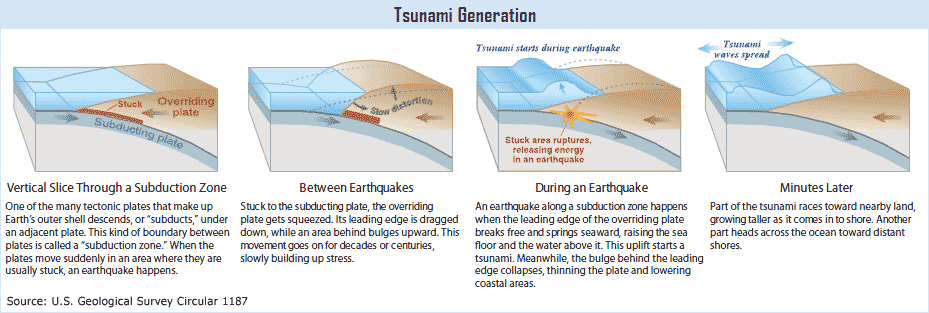The image is a set of four textbook-style, cutaway illustrations titled "Tsunami Generation," sourced from U.S. Geological Survey Circular 1187. The diagrams provide a detailed visual sequence of the process of tsunami formation at a subduction zone. The first illustration, labeled "vertical slice through a subduction zone," shows a cross-section where one tectonic plate descends beneath another, explaining how sudden movements cause earthquakes. The second, "between earthquakes," depicts the gradual deformation and stress buildup over decades or centuries, where the overriding plate gets squeezed, its leading edge dragged down while an area behind bulges upward. The third, "during an earthquake," illustrates the moment when the leading edge of the overriding plate snaps and springs seaward, raising the seafloor and the water above it, initiating the tsunami. The final image, "minutes later," shows the resulting tsunami waves, which grow taller as they approach the shore, while another part traverses the ocean toward distant coasts. The diagrams are vividly colored with blue for water, and gray and tan for tectonic plates, effectively illustrating the dynamic interactions between Earth's geological layers.